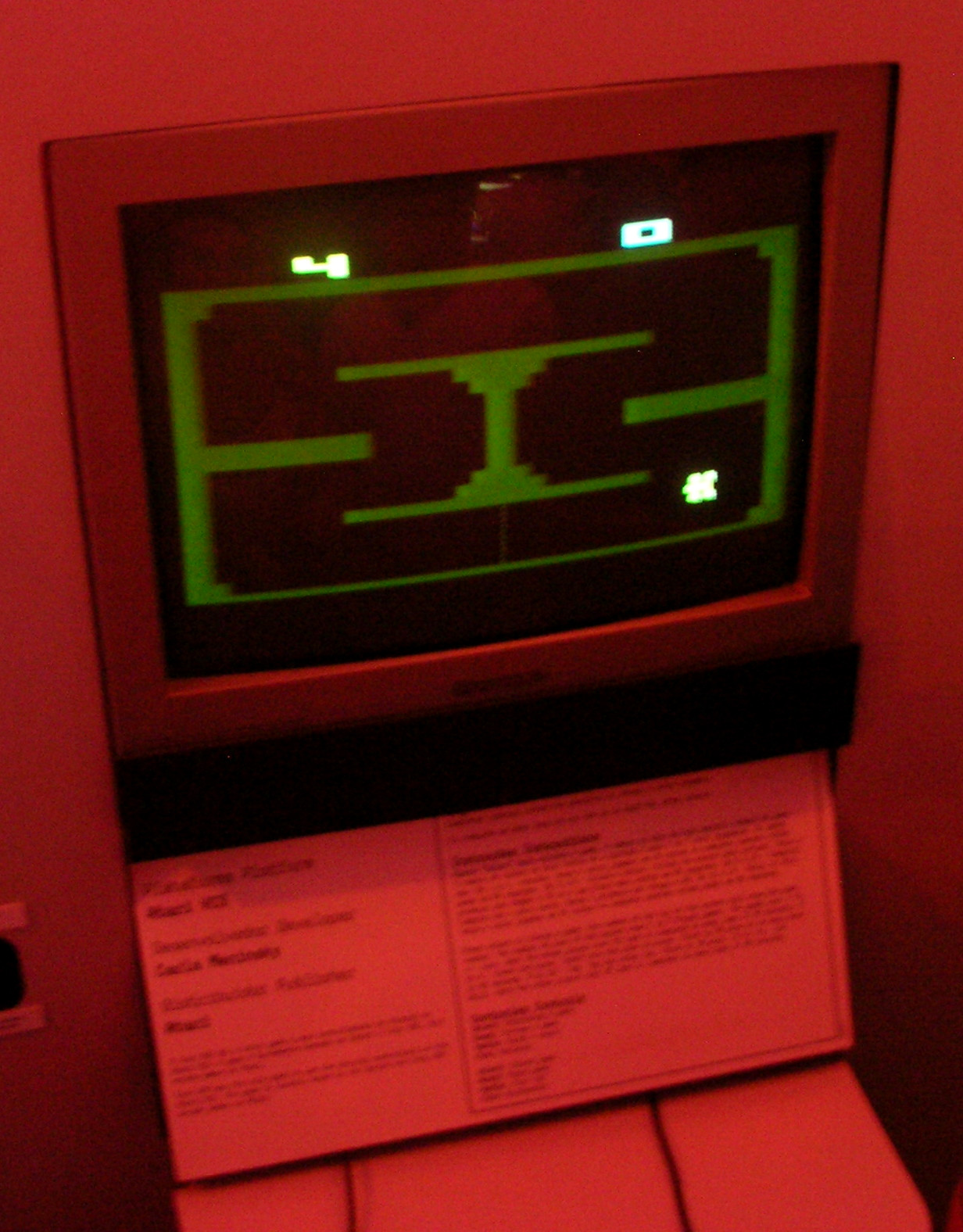The image features an old-style CRT television with a silver border, recessed into a wall and bathed in a red-tinted light that casts an overall red glow on the scene. The TV screen displays a retro video game characterized by simple, colorful graphics. Prominently featured on the screen is a green rectangle enclosing a symmetrical green hourglass-like shape, forming a rudimentary maze or track. Extending from the left and right sides of the rectangle are small beams. At the top of the screen, the score is displayed, with a '4' on the left and a '0' on the right. An irregular white blob is visible in the lower right of the screen, possibly representing a character or game object. Below the television, there is a plaque with black text that is not legible in the image, suggesting it might be an explanatory card, pointing towards a possible museum display of early video game technology or a store exhibit.